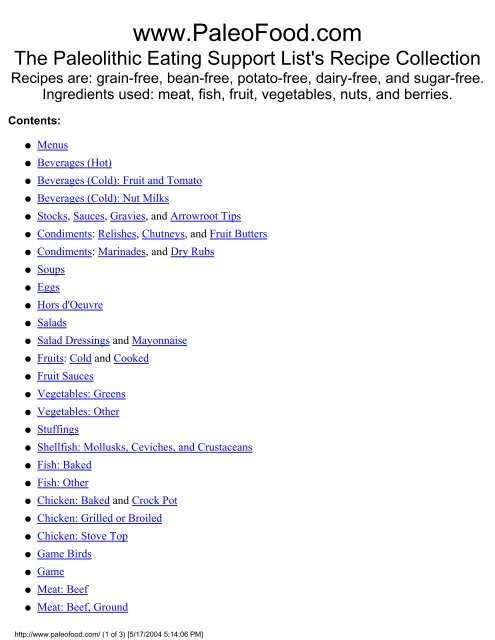A screenshot captures the homepage of PaleoFood.com, prominently displaying the site's name at the top. Right beneath the website’s title is the statement: "The Paleolithic Eating Support List Recipe Collection." This sets the tone for the content, indicating that the recipes adhere to a Paleo diet, characterized by the exclusion of grains, beans, potatoes, dairy, and sugar. Allowed ingredients include meat, fish, fruits, vegetables, nuts, and berries.

Following this introduction is a detailed list of approximately 25 categories of content available on the site, organized for easy navigation. These categories include: 

1. Menus
2. Beverages, hot
3. Beverages, cold (fruit and tomato)
4. Beverages, cold (nut milks)
5. Stocks, sauces, gravies, and arrowtips
6. Condiments, relishes, chutneys, and fruit butters
7. Condiments, marinades, and dry rubs
8. Soups
9. Eggs
10. Hors d'oeuvres
11. Salads
12. Salad dressings and mayonnaise
13. Fruits (cold and cooked)
14. Fruit sauces
15. Vegetables (greens)
16. Vegetables (other)
17. Stuffings
18. Shellfish, mollusks, ceviche, and crustaceans
19. Fish (baked)
20. Fish (other)
21. Chicken (baked and crockpot)
22. Chicken (grilled or broiled)
23. Chicken (stovetop)
24. Game birds
25. Meat (beef)
26. Meat (beef, ground)

Each category aims to provide a variety of recipes that align with the strict dietary guidelines of the Paleo diet, ensuring readers can find suitable options for every meal and occasion.